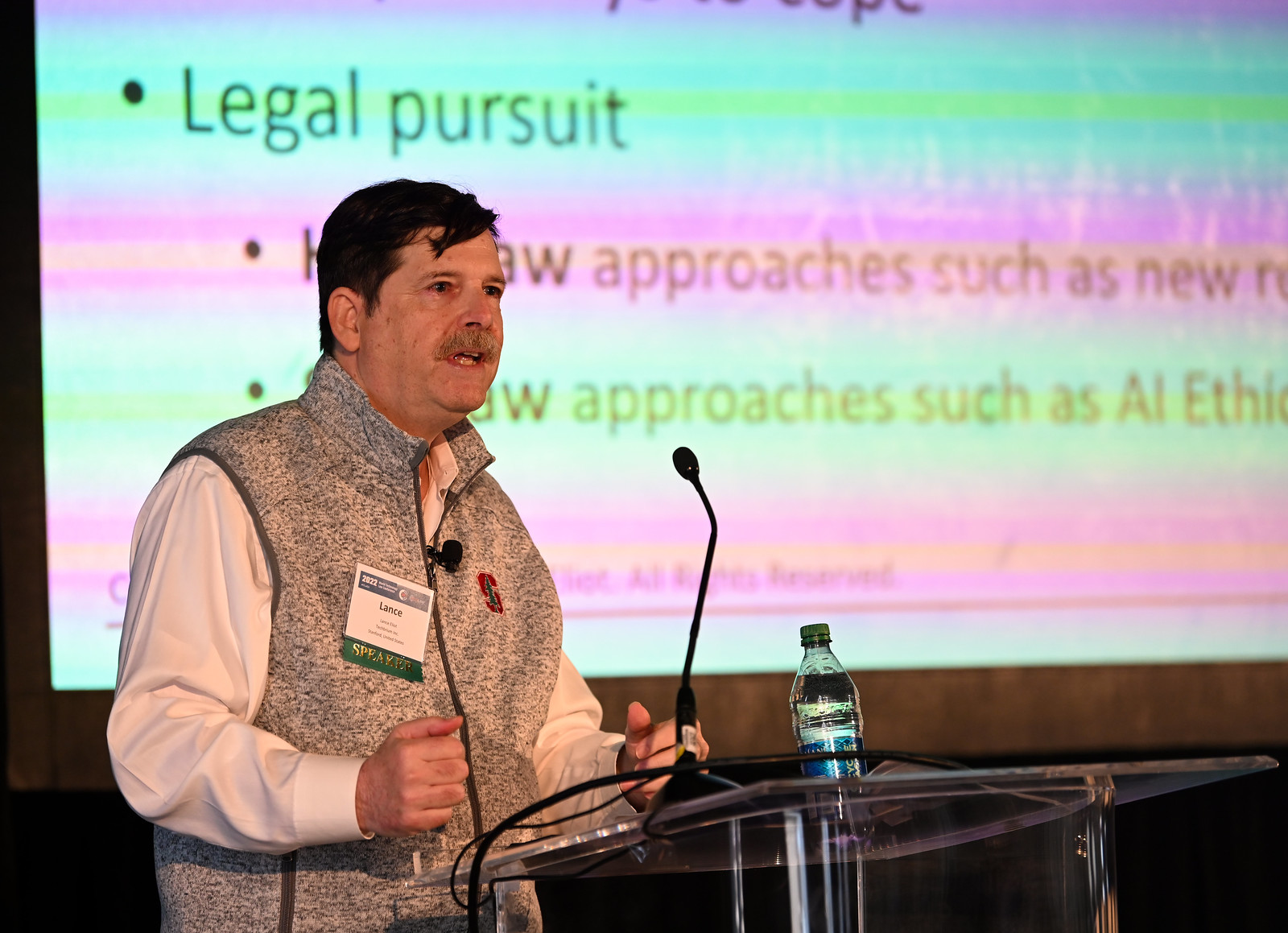The photograph captures a man named Lance, identifiable by his white, blue, and green nametag which includes the word "Speaker" beneath his name, who is addressing an audience from behind a podium. The podium, positioned towards the right side of the image, is made of clear plexiglass and houses a black microphone and a water bottle. Lance stands to its left, wearing a white shirt beneath a gray vest, and sports dark hair with a lighter-colored mustache. Behind him, occupying most of the background, is a large projector screen displaying a PowerPoint slide with a striped blue, green, and pink hue, perhaps due to color warping. Visible on the slide is black text, specifically the phrase "Legal Pursuit," along with partial phrases that include "Approaches Such As New" and potentially "Approaches Such As AI." The surroundings feature dark brown walls, reinforcing the focus on the man and the screen during his presentation.